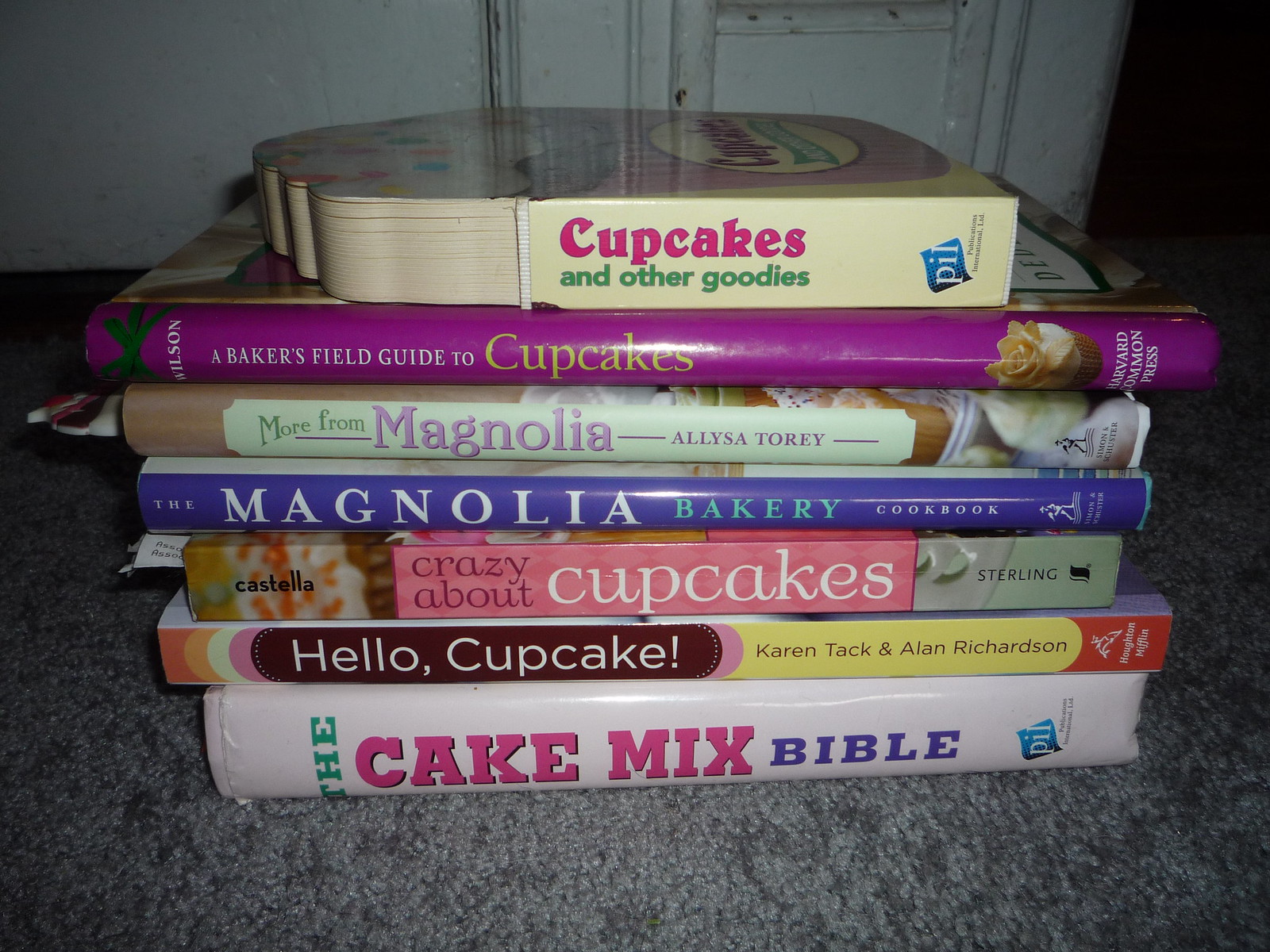The image depicts a stack of seven books neatly arranged on a blue carpet. The base of the stack is "The Cake Mix Bible," which has a distinct blue cover adorned with varied typography: "The" in green letters, "Cake Mix" in pink, and "Bible" in blue. Directly atop this lies "Hello Cupcake" by Karen Tack and Alan Richardson, featuring a bold white font on a yellow background for the title and black letters for the authors' names. Next is "Crazy About Cupcakes," where "Crazy About" appears in pink and "Cupcakes" in white. Above this stands "The Magnolia Bakery Cookbook," identifiable by its classic blue spine and white text. Following is "More from Magnolia" by Alyssa Torre, showcased with an enticing image of various pastries on the cover. Higher up sits "A Baker’s Field Guide to Cupcakes," marked by a visual of a cupcake on the cover. Concluding the stack at the top is a smaller book titled "Cupcakes and Other Goodies."